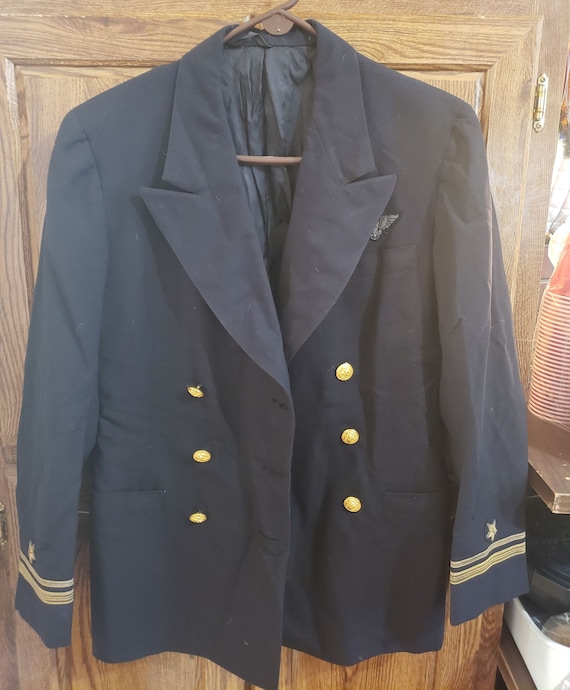In this photograph, a grayish-dark blue jacket is prominently displayed, hanging on a brown plastic hanger against a brown wooden door. The jacket, occupying the central position and almost 90% of the image, is neatly positioned to face forward. This garment features wide lapels and a double-breasted design with three gold buttons on each side. Distinctive gold stripes adorn the sleeves, each stripe featuring a single star in the middle. The jacket appears wrinkled, indicating it hasn't been pressed. The setting appears to be a closet, with shelving visible next to the door.